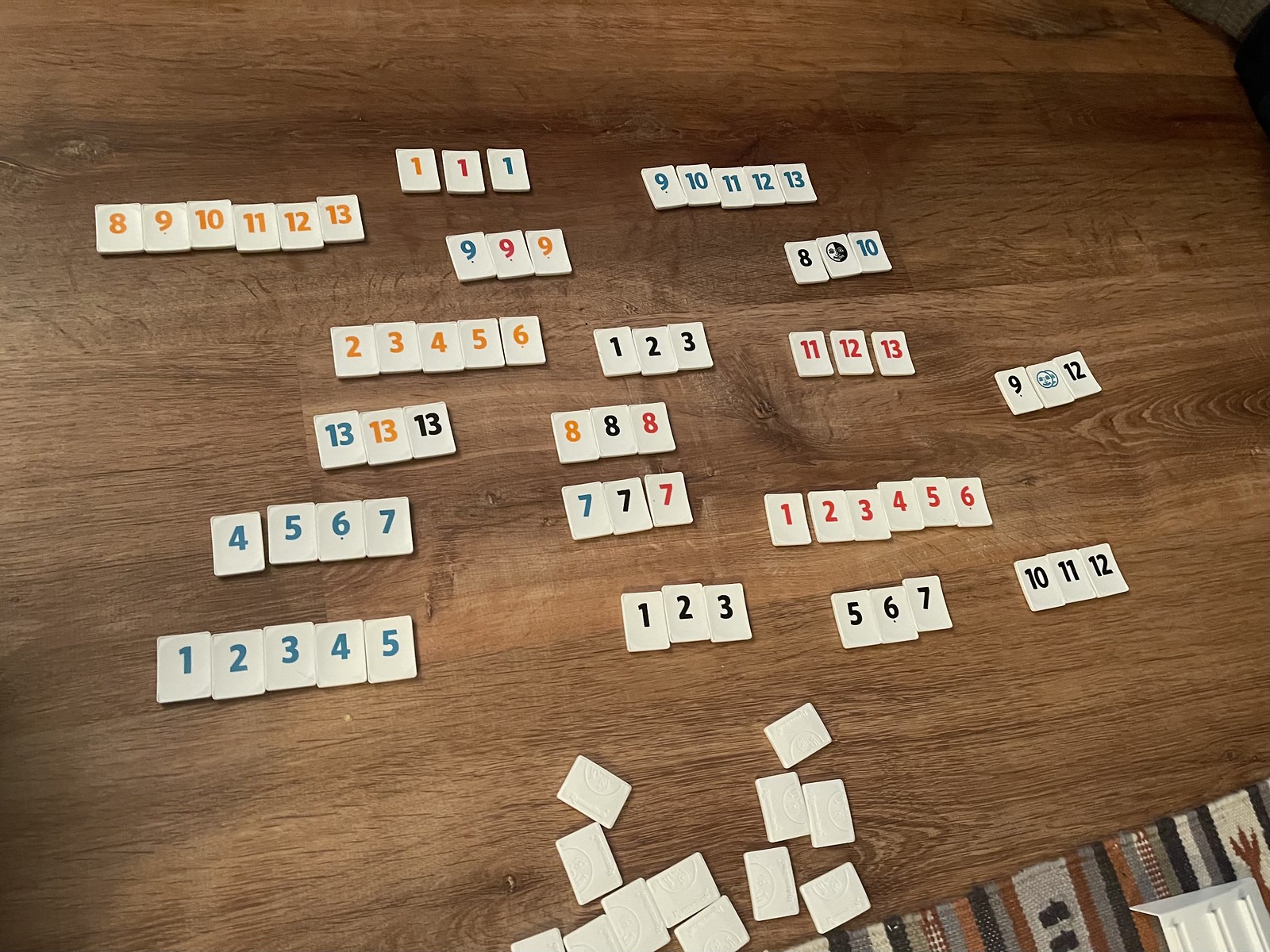This image showcases a collection of numbered tiles, likely used for a strategic game, arranged in a visually organized manner on a dark brown wooden floor. The fine grain of the wood runs horizontally, adding a rustic charm to the setting. At the bottom of the image, some tiles lie face down, revealing their thickness and the shadows they cast, confirming they are indeed tiles and not playing cards.

The backdrop features an Indian-styled woven blanket, which adds a touch of cultural richness and warmth to the scene. The tiles are meticulously grouped by color and sequence. At the top, there are three '1's in different colors. Below them, a sequence from 8 to 13 in orange, followed by a green sequence from 9 to 13. Nearby, there are three '9's, each in a distinct color, indicating a possible set.

Further down, sequences from 1 to 6 in red, 1 to 5 and 4 to 7 in green, as well as 1 to 3, 5 to 7, and 10 to 11 in black, can be seen, showing a variety in grouping patterns. Additionally, sets of three '8's, three '7's, three '13's, and a couple of 2 to 6 tiles in orange are also present.

The arrangement hints at a game where grouping by sequence or color is essential, though the exact nature of the gameplay remains unclear. The careful organization and vivid colors make the image not only informative but visually engaging.